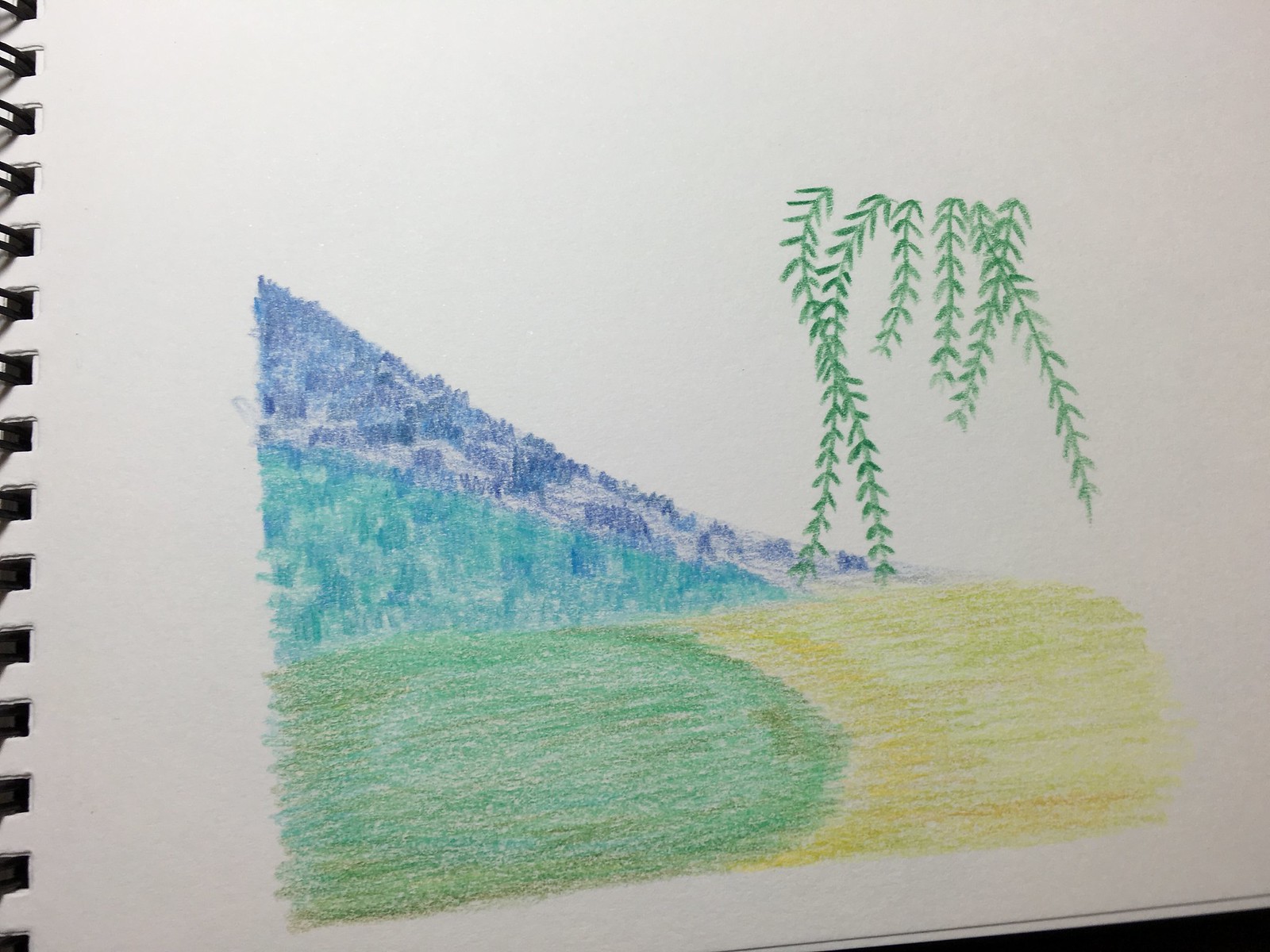A detailed and descriptive caption for the image could be:

"A detailed sketch in a ring-bound sketch pad showcases a layered landscape. Starting from the bottom, a green area resembling a field is depicted, flanked by a yellow section to the right that hints at a crop field. Above these, a triangular blue area with sparse vegetation slopes upward, giving way to an even steeper and darker blue section, also adorned with plant growth. In the top-right corner of the image, surreal vines or leaves hang mysteriously from the sky, with no visible connection to any plant or tree, creating an intriguing and otherworldly scene."